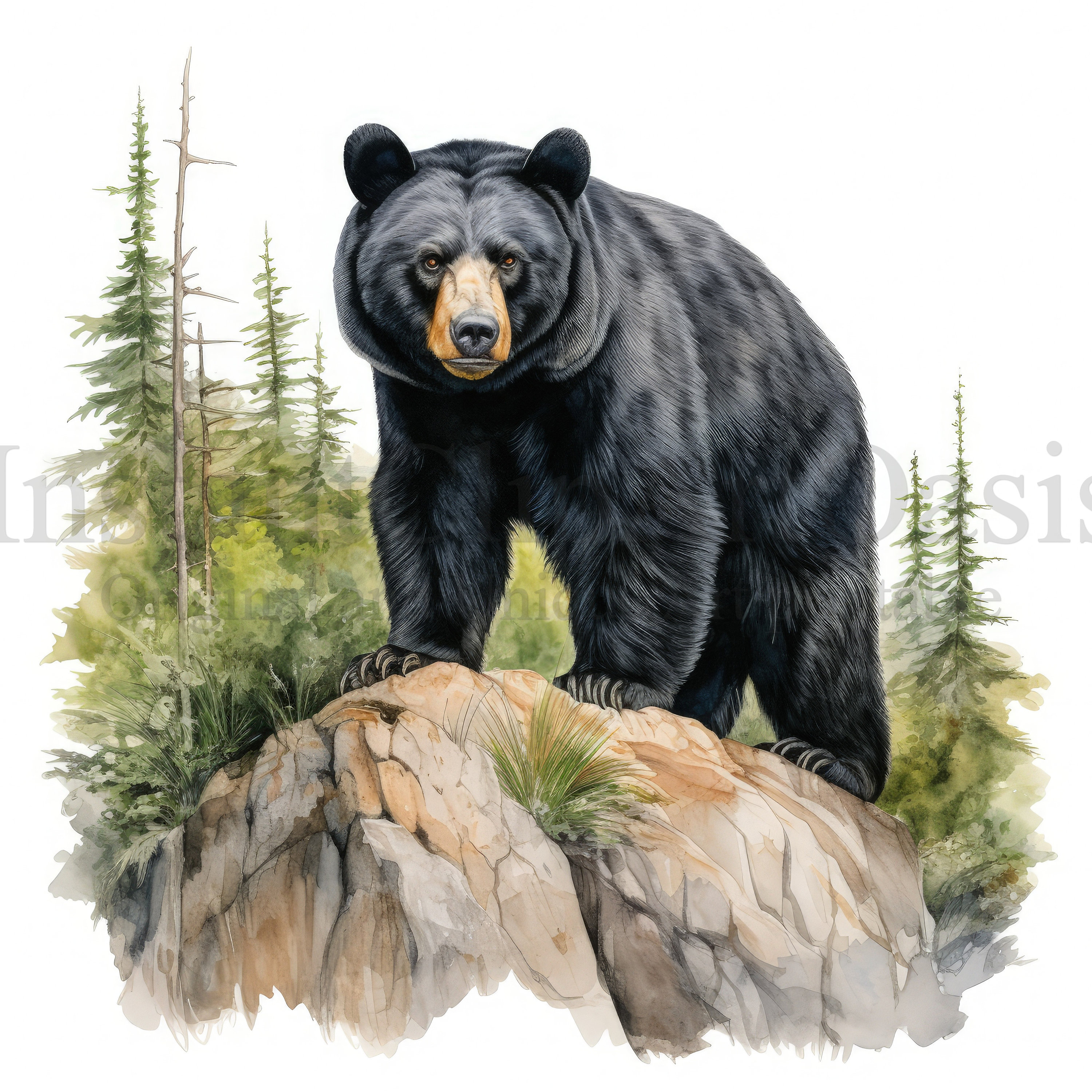This detailed painting captures a striking black bear standing prominently on a large, tannish-brown rock, which has cracks and tufts of grass sprouting from its crevices. The bear, with its realistic and detailed black fur interspersed with hints of silver, boasts a distinguishing light brown snout and sharp, formidable claws gripping the rock. The bear's commanding presence is emphasized by its intense gaze directed straight at the viewer. Surrounding the bear, a lush forest landscape unfolds with green trees, some of which have leaves indicative of springtime, while others are barren, resembling lifeless sticks. The background blends into a verdant blur, enhancing the sense of wilderness and depth in the scene.